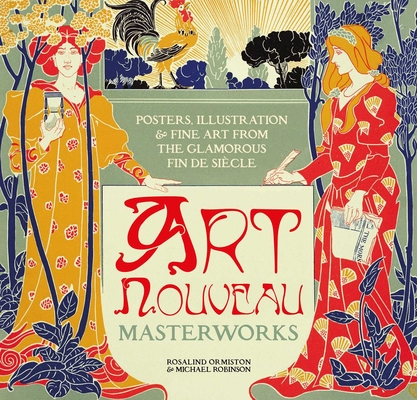The image, presented in a square orientation, serves as a cover or poster combining vibrant and highly stylized artwork with descriptive text. At the top, the text reads "Posters, Illustration, and Fine Art from the glamorous Vin de Cecil." Below this, in a more ornate font, it states, "Art Nouveau Masterworks," and lists the authors as Rosalind Ormiston and Michael Robinson. Dominating the visual are two figures: a man on the left and a woman on the right, both illustrated in exaggerated, cartoonish styles. The man, adorned in a yellow floral robe and a turban-like hat, stands out against a red and blue color palette. In the middle, a rooster struts across the scene, adding dynamic movement. On the right, the woman wears a striking red dress embellished with a paper fan pattern. Both figures are set against intricate backgrounds of vines and bushes, incorporating a limited yet vivid color scheme dominated by reds, yellows, blues, teals, and greens. This detailed composition reflects the elegant and colorful nuances of the Art Nouveau era.